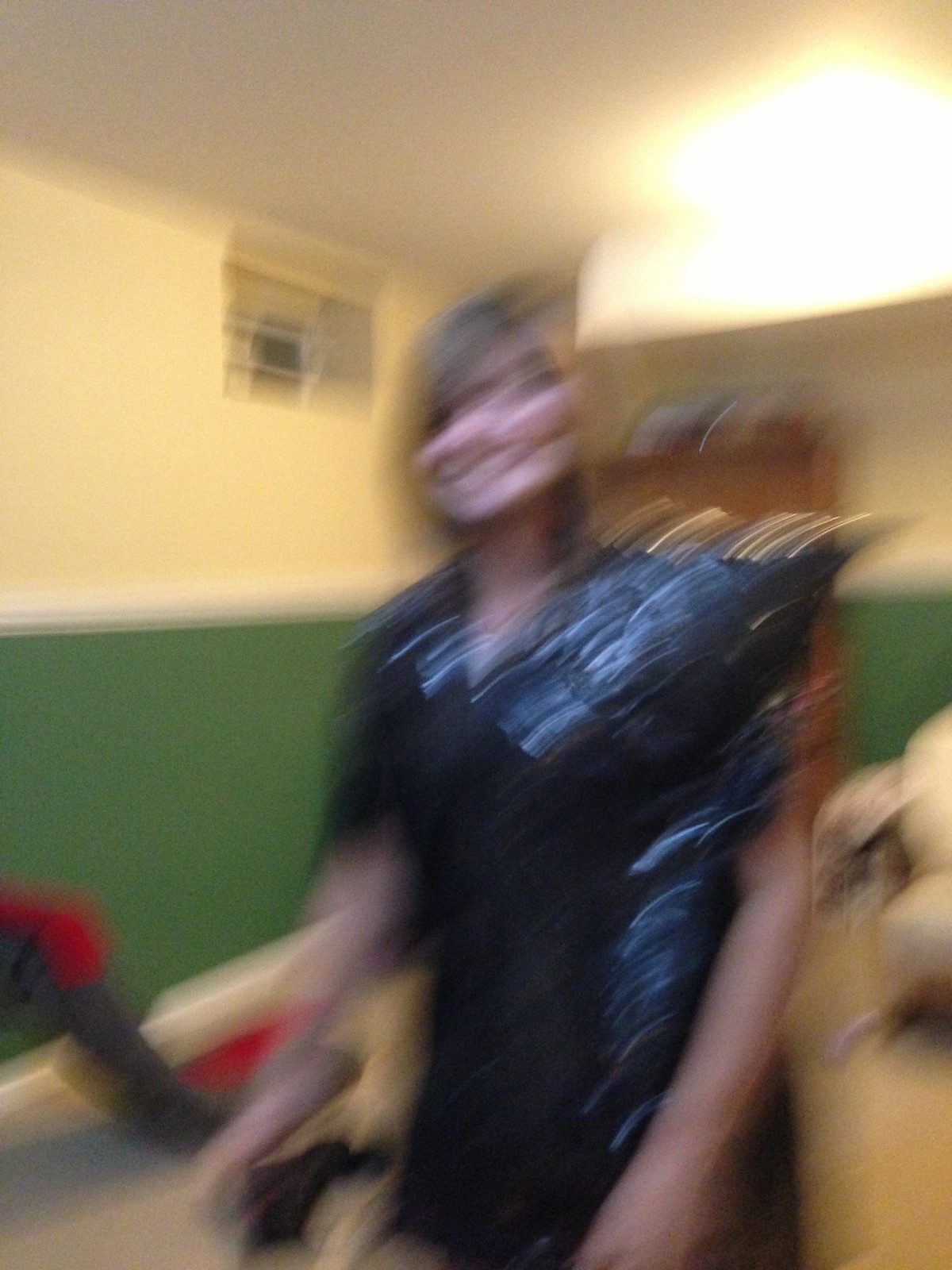In this blurry image, we see a corner of a room that resembles a corridor in a school or hospital. The walls are divided into two sections: the lower part is covered with a green panel and is topped with a white rail, while the upper portion is painted cream. Near the center, there's an unclear feature that appears to be either a picture or a recessed area. In the foreground, there is a figure dressed in a short-sleeved or sleeveless blue garment, with their arms extended forward as if they are pushing an object, possibly a trolley. Behind the figure, there is an indeterminate white object, which is unlikely to be an animal given the indoor setting. The person's face is indistinct, making it impossible to determine their gender.